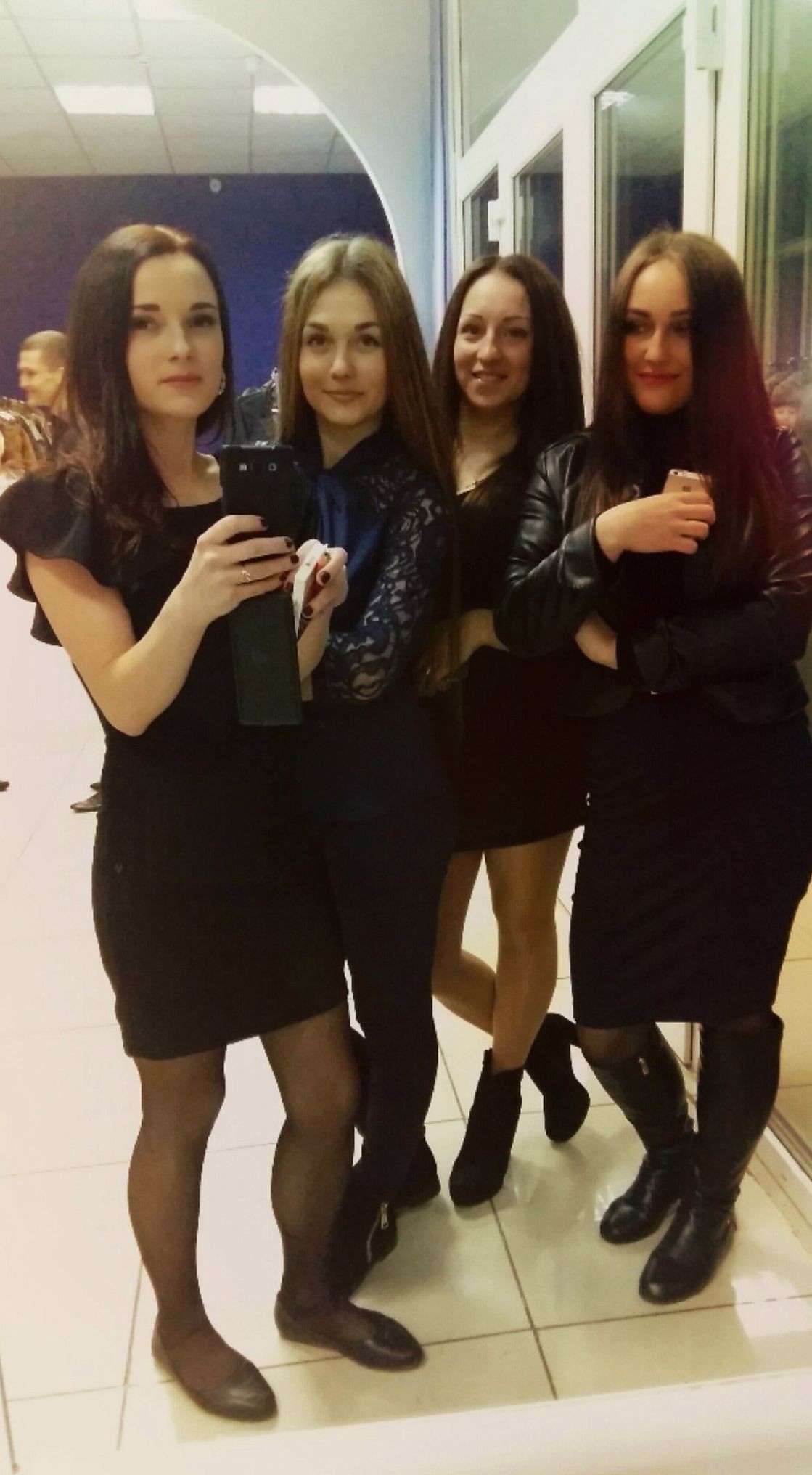In this vertically aligned rectangular image, four young women are standing and posing together, seemingly taking a group selfie in front of a mirror with a cellphone. Each woman has long dark hair and is smiling at the camera. They are all wearing different variations of black attire. The woman on the far left is in a black dress with black stockings and flat shoes, and she is holding the phone. Next to her, a woman wearing a blue lace top paired with dark pants and zippered boots stands. The third woman is dressed in a short black dress with high-heeled boots, while the woman on the far right sports a black leather jacket, a long black dress, black tights, and knee-high leather boots. They are standing on large white tiles with visible grout lines, within a room lit by fluorescent lights in a square-tile ceiling. Behind them, an arched doorway leads into a room with a large dark blue wall. In the background, other people can be seen, including a man with short hair walking towards the left, indicating that this might be some sort of event or gathering.